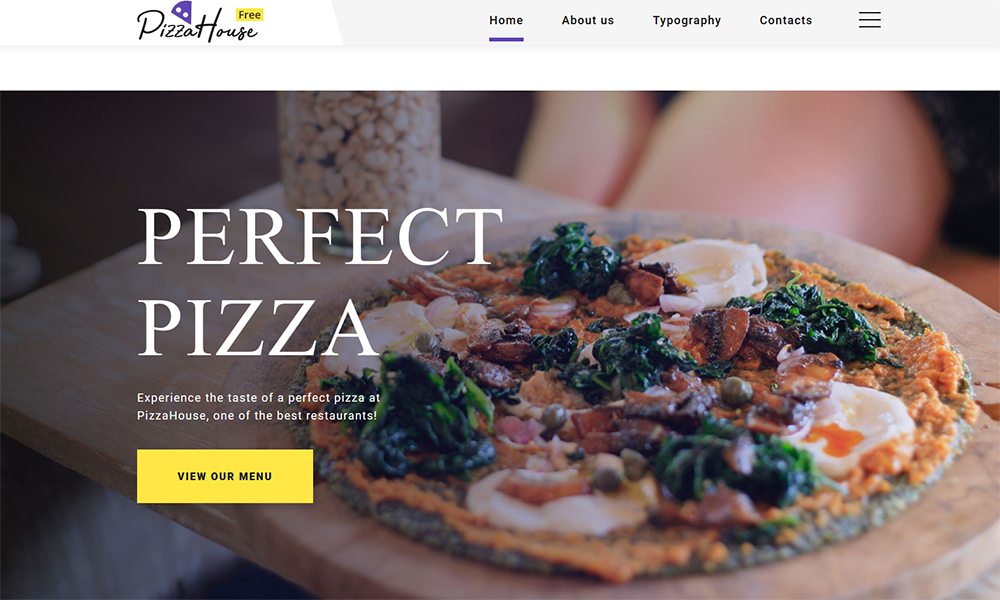This is a left-to-right horizontal image, likely a screenshot taken from a computer or smartphone, showcasing a restaurant's website, specifically a pizza place. The website has a predominantly white background. 

At the top left corner, the logo "Pizza House" is displayed, with a small, purple slice of pizza featuring two white circles, diagonally jutting out from the letter "A". Next to it, a yellow box with black letters reads "Free". On the top right side is a gray box featuring the word "Home" in black, underlined in purple, accompanied by links labeled "About Us", "Topography", and "Contacts", with three horizontal black lines suggesting a menu.

The central part of the image highlights a photograph of a pizza placed on a rustic brown wooden tray. This pizza is adorned with various colorful vegetables, indicative of a vegetable pizza. The background of the image blurs out, hinting at what appears to be a person's legs, directing focus to the pizza.

Overlaying the image, bold white uppercase text announces "PERFECT PIZZA", with a subtitle in white saying "Experience the taste of perfection at Pizza House, one of the best restaurants." Below this is a yellow rectangular box with black text inviting viewers to "View Our Menu".